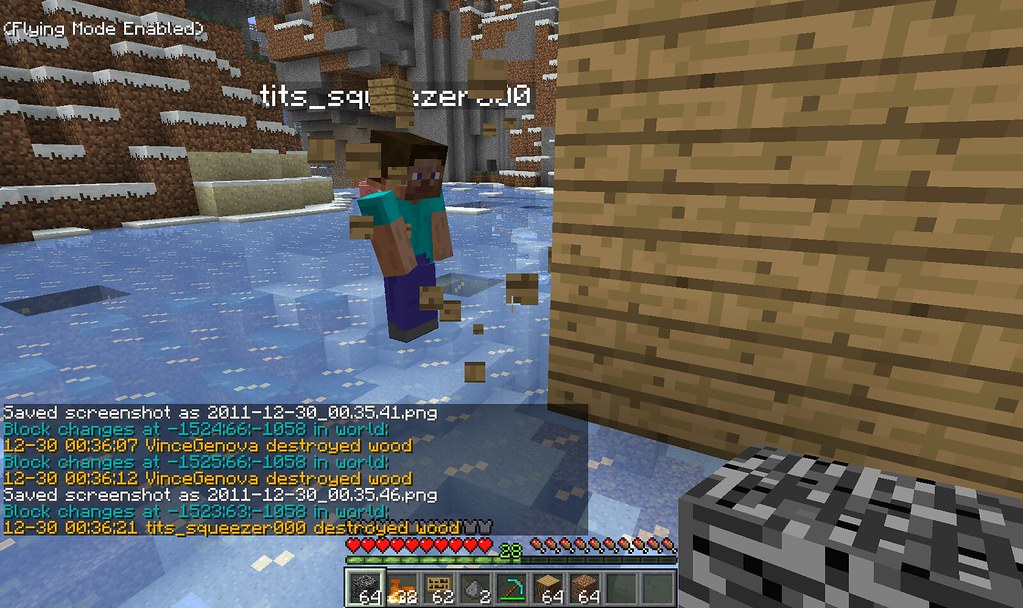A still screenshot from the game Minecraft features a central blocky character with dark hair and skin, dressed in a teal shirt and dark blue pants. The character stands atop blue water, seemingly defying gravity. In the background to the left, a towering hill or mountain is visible. Facing a wooden wall to the right, the character’s name, "titsqueezer000," is displayed prominently on the screen. The top left corner indicates that "flying mode" is enabled. On the bottom left, some text appears to record in-game actions: "saved screenshot as [filename].png," along with repeated lines "vintgenova destroyed wood." At the screen's bottom, different materials and quantities are shown along with a row of hearts, likely indicating the character’s health points. Every element adheres to the distinct blocky aesthetic of Minecraft.